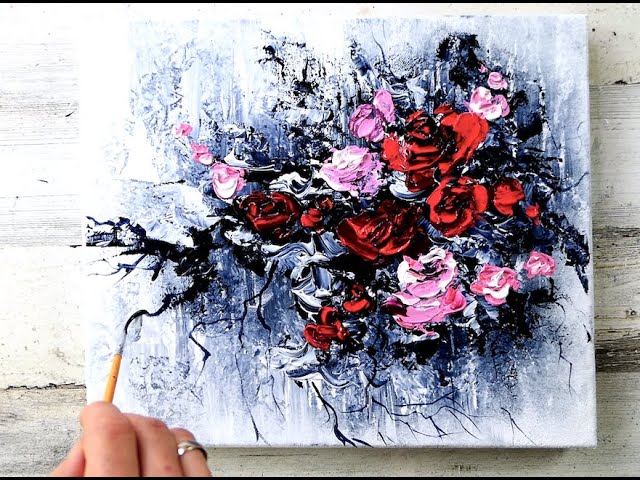The image depicts an acrylic-on-canvas painting, its white canvas stretched over a six-inch by six-inch wooden frame. The central focus is a large, detailed cluster of roses in various colors, including dark red, light pink, and blackish gray. Black vines intertwined around the roses enhance the overall composition, adding a dark, intricate contrast against the flowers' vibrant hues. The background features subtle streaks of white and blue, giving a scattered, ethereal effect.

In the lower left corner, the artist's hand is visible; three fingers delicately hold a yellow paintbrush with a silver metal ferrule, intricately painting one of the black vines. The artist wears a silver ring on the fourth finger. The photograph is set on a backdrop of faded wooden planks, providing a rustic contrast to the vividness of the painting. The image captures the blend of detailed realism and abstract elements, merging dark and light tones in a harmonious yet striking composition.